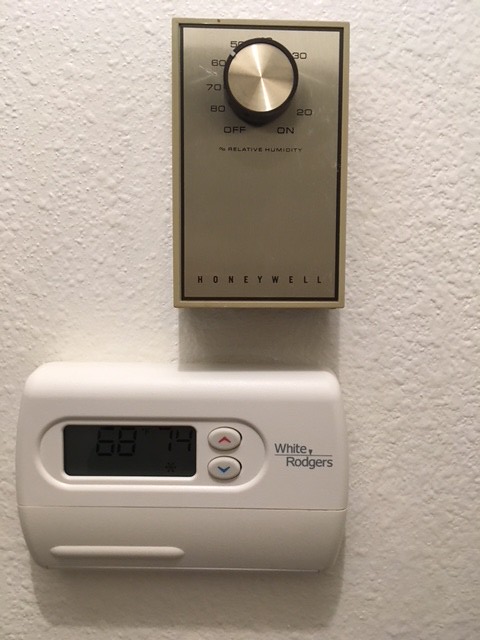The close-up image captures a section of a white wall adorned with two thermostats. The first thermostat, a rectangular device positioned with its longer sides horizontal, boasts a metallic gold and silver finish. The Honeywell brand name is prominently displayed in black at the bottom of this thermostat. A dial near the top is encircled by temperature markings starting from "Off" in the bottom left corner and ascending through 80, 70, 60, 50, skipping higher values to 30, and finally a gap before 20 on the far right. The "On" indicator is located in the bottom right corner. 

Below this device, a second thermostat, also rectangular but oriented vertically, features a clear digital display reading "68" and "74". The brand "White Rogers" is written to the right of the screen. This thermostat includes two distinctive white buttons: one with a red upward arrow and the other with a blue downward arrow. Below the buttons, there's a partially opened flap, hinting at additional controls that can be revealed by flipping it down.